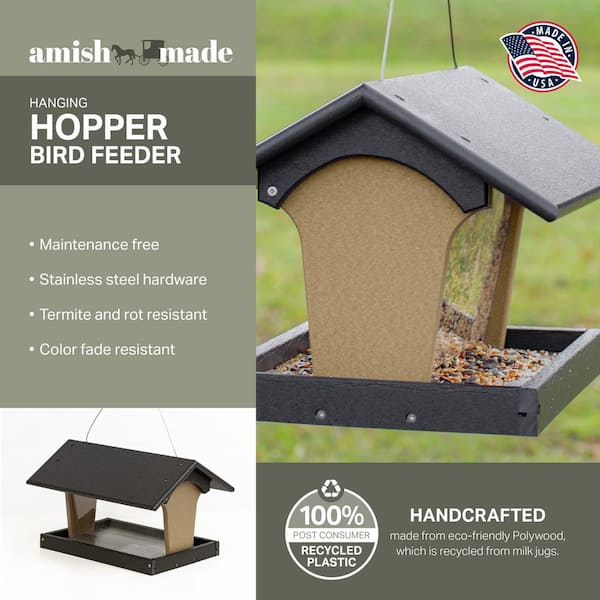This image is an advertisement for an Amish-made, hanging hopper bird feeder, featuring a highly detailed and descriptive presentation of its features. The bird feeder is presented with a natural colored wood side, a deep green roof, and a deep green tray at the bottom. Its open design includes glass sides and strings for easy suspension, allowing seeds to spill out onto the tray. Highlighted features include maintenance-free construction, stainless steel hardware, resistance to termites and rot, and color-fade resistance. Crafted from eco-friendly polywood, the feeder is made from 100% post-consumer recycled plastic, specifically recycled from old milk jugs. The advertisement emphasizes its handcrafted quality and American origin, with a "Made in the USA" badge paired with an American flag. The detailed depiction shows the feeder both empty and in use, showcasing its practicality and aesthetic appeal.